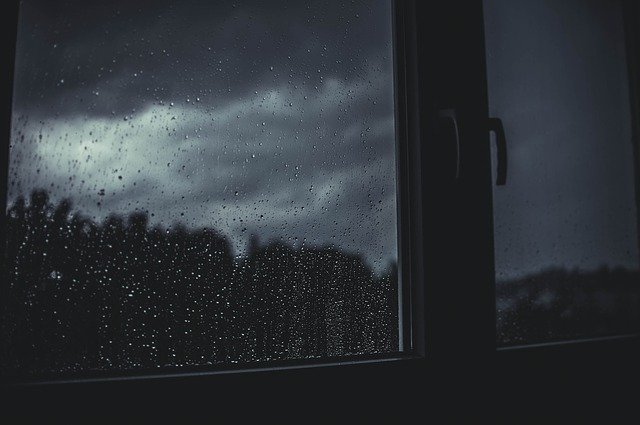This photograph, tinged with an eerie and somber atmosphere, captures the view from inside a dimly lit room through large glass doors or a window. The setting appears to be during night or the very early hours of the morning, adding to the overall dark and mysterious tone. Rain falls heavily, leaving raindrops and condensation on the glass pane, and outside the window, dark, heavy clouds obscure much of the scene. The haziness creates a sense of vagueness, obscuring details and making it challenging to discern whether the backdrop features a city skyline or a cluster of trees. The grayscale appearance of the photograph further enhances the eerie and surreal quality of the scene.